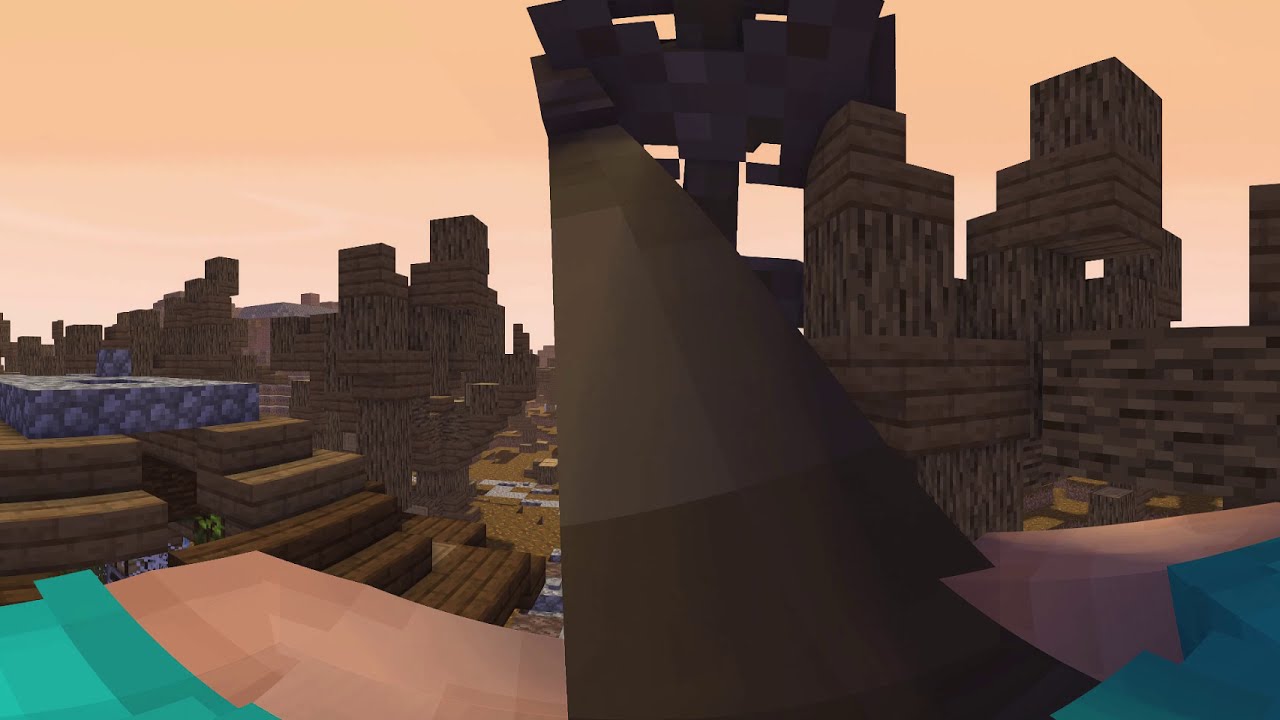This is a detailed screenshot from a Minecraft-like game featuring highly blocky and cartoonish graphics. The scene captures a character with white hands wearing a turquoise blue shirt, seemingly holding a weapon or an object. The backdrop reveals an intricate landscape resembling an old medieval town constructed with brown and tan bricks. Towering wooden pillars, rocks, and blocks suggest a fortified base or fortress with multiple columns and staircases. The landscape is rich in color with dark and light browns, accented by patches of pink, aqua blue, lavender, and purple, contributing to the vibrant atmosphere. The sky is an orange hue, indicative of a near-sunset setting, further enhanced by clouds. The image, taken from a high vantage point, overlooks a courtyard devoid of human-like figures, reinforcing the sense of quiet and intricate design in this expansive, outdoor digital world.